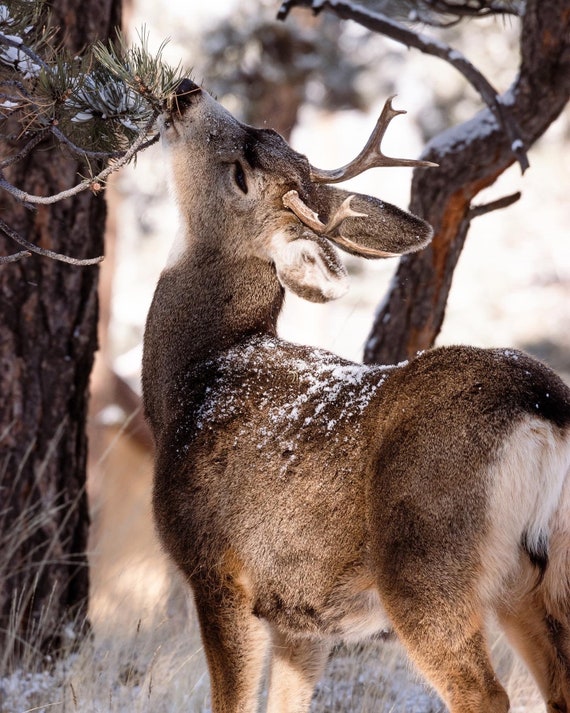In this detailed wildlife photo taken during the daytime, a young male deer, identified by the small growth of antlers on the sides of its head, is captured nibbling on the needle-like leaves of an evergreen tree in a winter forest. The deer, with its light beige fur, is lightly dusted with snow on its back, enhancing its cute appearance. Snow also gently covers the branches and the forest floor, emphasizing the wintry setting. The scene is serene and natural, showcasing the deer's instinctive behavior as it reaches up to feed on the branches amidst the quiet beauty of the snowy woodland.